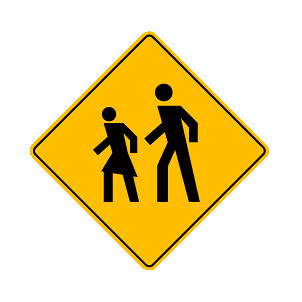The image depicts a yellow, diamond-shaped street sign with a black border running along the edge. At the center of the sign, two stick figures—a female wearing a skirt and a taller male—are illustrated, appearing to walk from right to left. The figures have their legs positioned as if in mid-step and arms raised, with the heads separated from their bodies, and neither figure has feet. The sign is specifically designed to indicate a school crossing area, highlighting the imminent presence of schoolchildren potentially crossing the street.